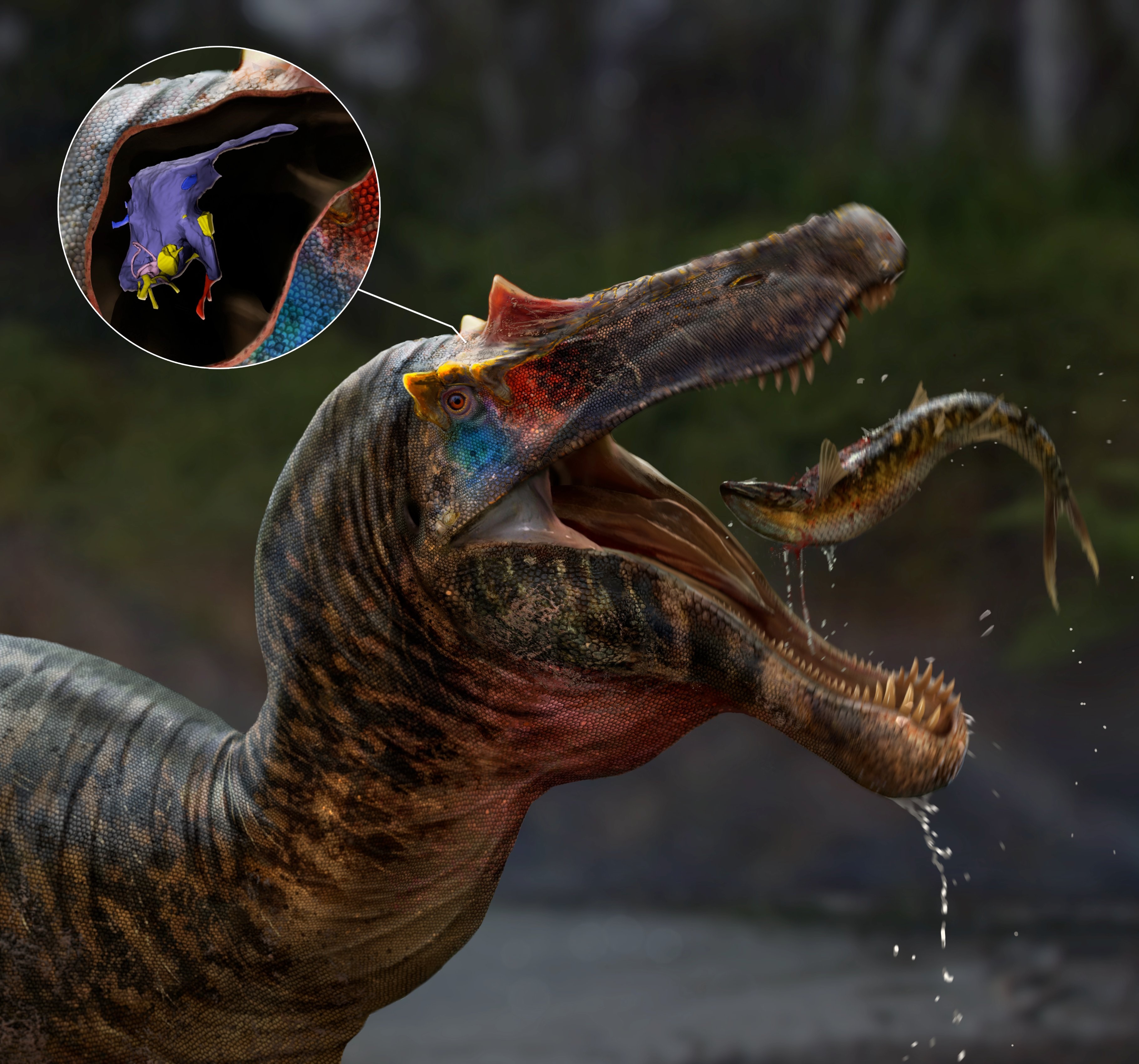A digital image showcases a prehistoric-looking reptile, remarkably lifelike, set against a blurred, mottled gray and green backdrop, resembling a riverside with vegetation. The reptile’s detailed head is positioned in the lower left of the image, facing a 2 o'clock direction with its long, narrow mouth wide open, revealing approximately 100 yellow, sharp teeth. Center to the composition, it appears to be in the act of catching a slender, brown fish mid-air, which is flopping as though it were just plucked from water, evidenced by dribbles of water falling from the reptile's mouth. The skin of the reptile is a smooth, matte, scaly texture, predominantly dark olive green with lighter beige stripes on its back, and a bronzed, golden underbelly. Distinguishing features include blue and red coloring around its eyes, notably highlighted by tiny spikes above them. An inset circle located at the 10 o'clock position zooms in on a portion of the head, focusing on the eye—depicted with a purple iris speckled with yellow, outlined against an off rust-red background with gray scaling.